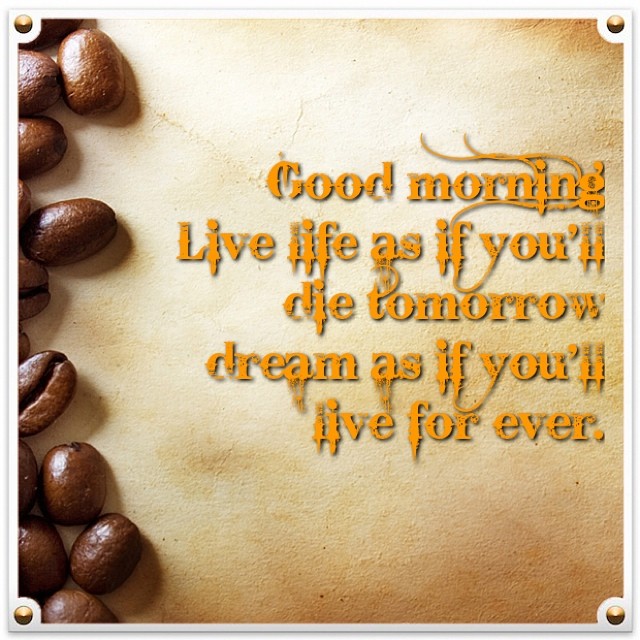The image is a digitally generated graphic with a whitish gray rustic background, featuring an intricate design. On the left, a small vertical row of brown coffee beans is displayed, some showing the familiar central line. The square image is bordered by a white frame with golden circles in each corner, resembling screws or nails that give the impression of the poster being tacked up. Centered on the right side, in fancy and stylish yellow-orange text, is the inspirational quote: "Good morning, live life as if you'll die tomorrow, dream as if you'll live forever." The overall composition combines the earthy tones of the coffee beans with the vibrant, creative typography for a visually engaging design.